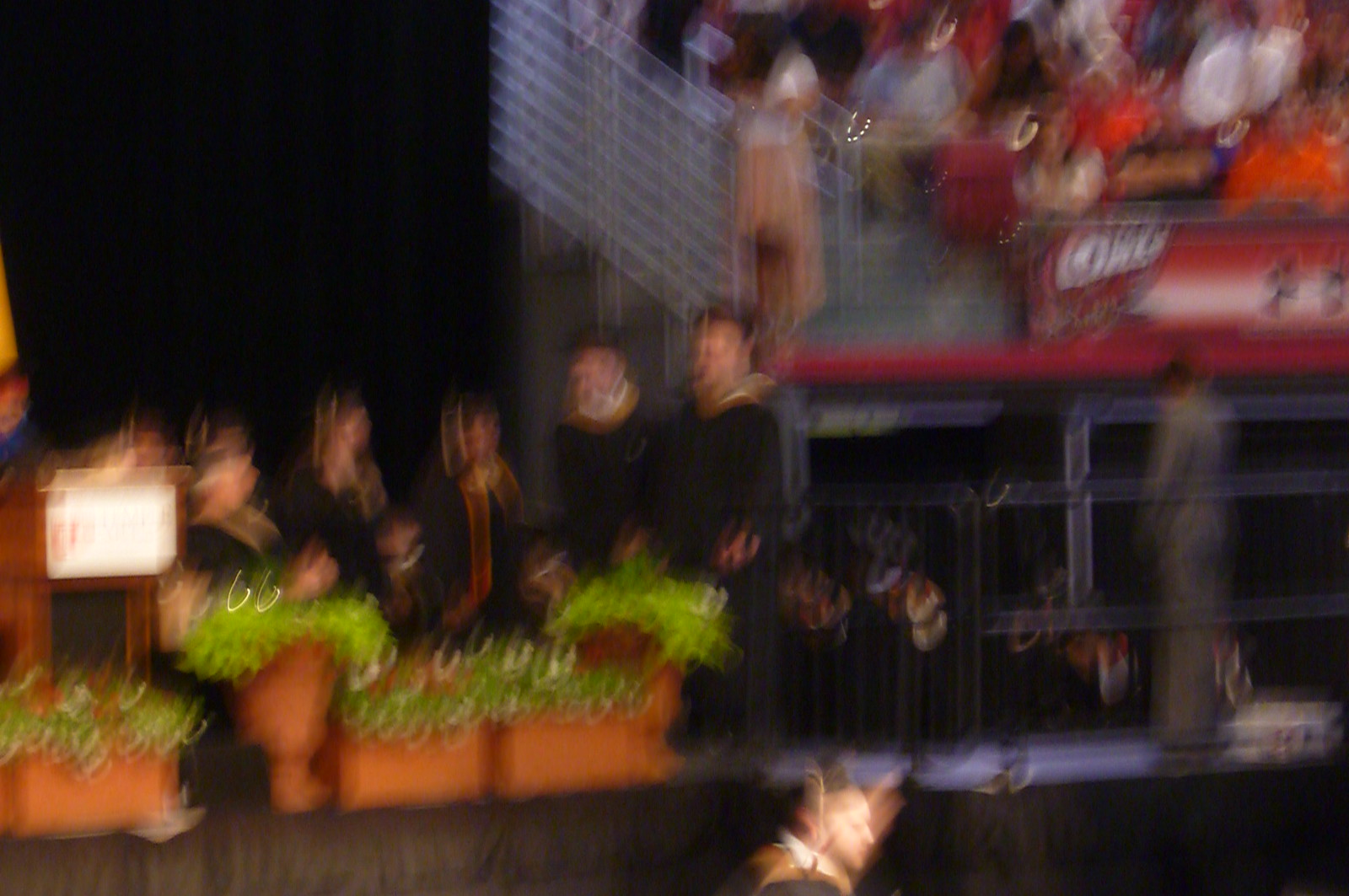A horizontally rectangular image, though extremely blurry and marked by motion-induced streaks of light on the left half, captures the scene of what appears to be a graduation ceremony. The indistinct shapes of several terracotta-style planters, filled with green plants, can be discerned at the forefront, seemingly positioned on or near a stage. Behind these planters stand several individuals clad in black gowns, a recognizable hallmark of graduation attire, who are aligned side by side. To the right, stretching upwards, faint outlines suggest the presence of bleachers, under which additional people stand, contributing to the celebratory atmosphere.